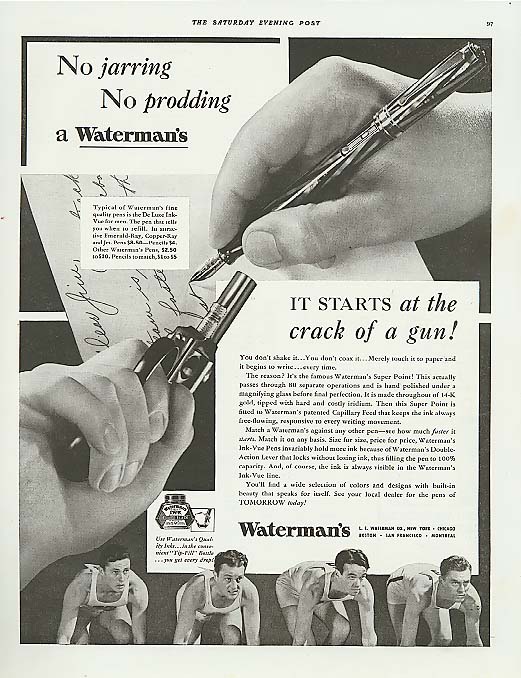In this vintage black-and-white advertisement for a Waterman's pen, the central focus is a right hand elegantly writing a letter with a Waterman's pen, symbolizing precision and quality. Below and to the left, a left hand holds a small gun, adding a dynamic contrast with an aura of traditional elegance juxtaposed against a sudden, sharp action. At the top left, bold text reads, "No jarring, no prodding, a Waterman's," emphasizing the pen's smooth performance. The phrase "it starts at the crack of a gun" is prominently featured in a large square at the bottom right of the image, drawing a parallel between the pen's reliability and the instant start of a race. At the bottom, four male track runners in tank tops crouch at the starting line, looking to the right, ready to spring into action. The composition suggests a seamless blend of meticulous craftsmanship and the exhilarating rush of competition, characteristic of high-end marketing from the 1950s.